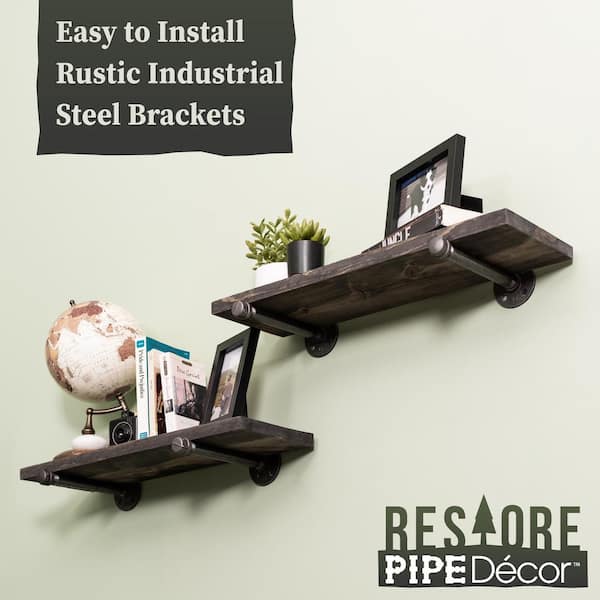The professional photograph features a minimalist design with two floating shelves affixed to a white wall, each supported by rustic industrial steel brackets that resemble cast iron pipes. The shelves, made of dark brown wood, are arranged in a square-frame format. The lower shelf holds a collection of items including a multi-colored globe (red, brown, yellow, and white), several books, and a black picture frame. The upper shelf displays two potted plants with green leaves; one pot is white and the other black, alongside another black photo frame placed on a book. In the upper right-hand corner of the image, a black rectangle with white text promotes the product as "easy to install rustic industrial steel brackets." In the lower right-hand corner, the Restore logo is showcased, with "Restore" spelled out in green and the 'T' stylized as a tree, accompanied by the words "Pipe Decor" in white text on a dark gray background. This clean, organized layout emphasizes the seamless blend of industrial and rustic styles, ideal for modern home décor.